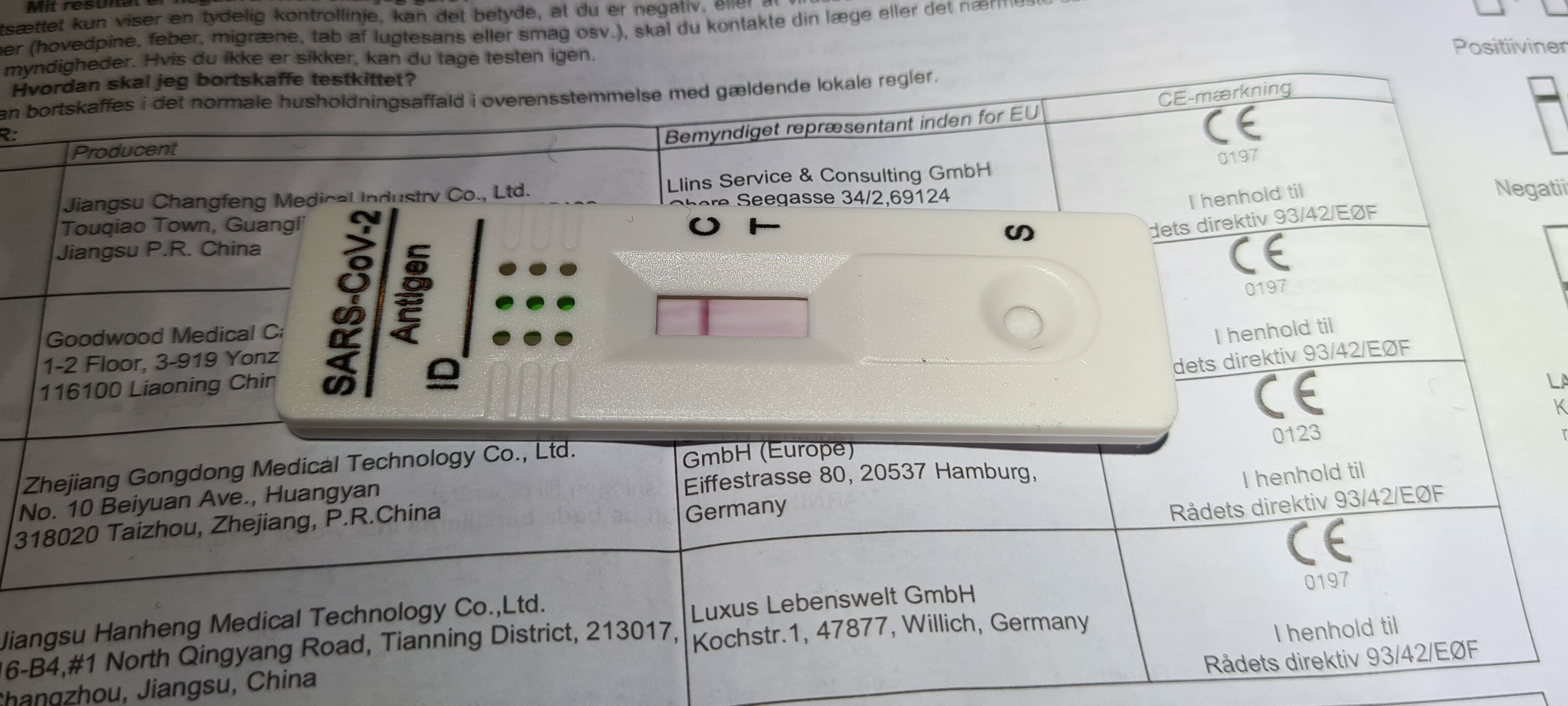This is a highly detailed photograph of a rapid COVID-19 antigen testing kit. The device, a rectangular off-white plastic apparatus, prominently displays the text "SARS-CoV-2 Antigen" at the top. Below this, there's a designated area labeled "ID" for an identification number, which is currently blank. On the far right of the device, there's a marked sample port labeled with an "S." 

In the central recessed area, you can see the "C" (control) and "T" (test) markings. The control line, marked by a stripe at the "C," is visibly prominent, indicating the test's validity. Conversely, there is no line at the "T," suggesting a negative test result for SARS-CoV-2 antigens.

The device is placed atop an instructional manual, printed in multiple languages. The manual includes the terms "medical technology," the CE logo, and various usage instructions. In the upper right corner of the manual, there are simple profile diagrams that illustrate the interpretations of positive and negative test results, aiding the user in understanding the tester.